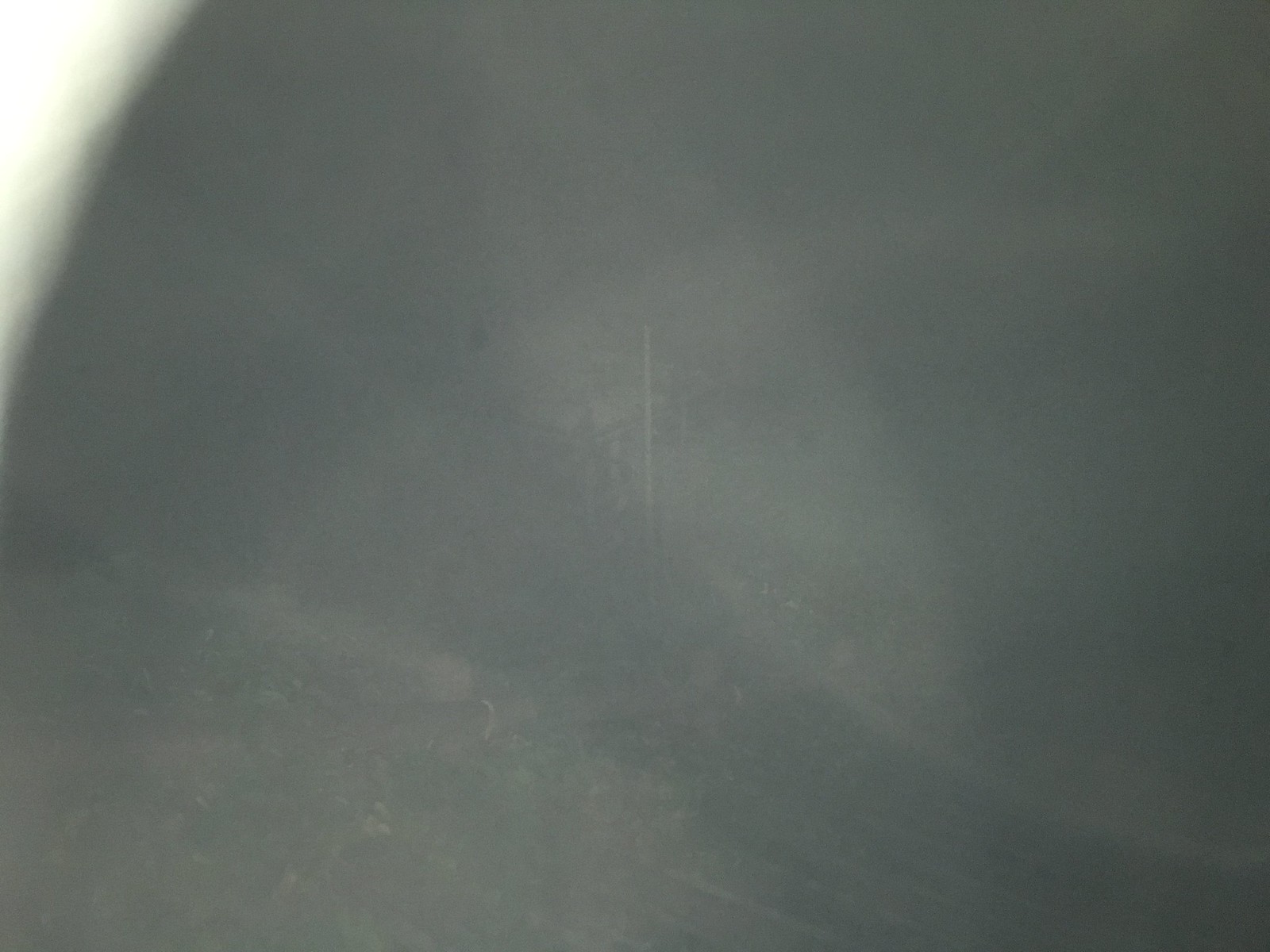This photograph is a heavily overexposed, indistinguishable color image primarily consisting of flat gray tones with occasional hints of light yellow. The scene seems to have been captured outdoors with a flash, resulting in significant reflection and overexposure. The top left corner of the image is completely washed out, while the rest of the photograph displays subtle gradations of gray. A circular arc of bright light extends from the bottom left corner to the top right quadrant, creating a petal-shaped pattern with varying hues. There are no discernible objects or details in the blurry, possibly misprinted photo, making it appear as a photographic anomaly.